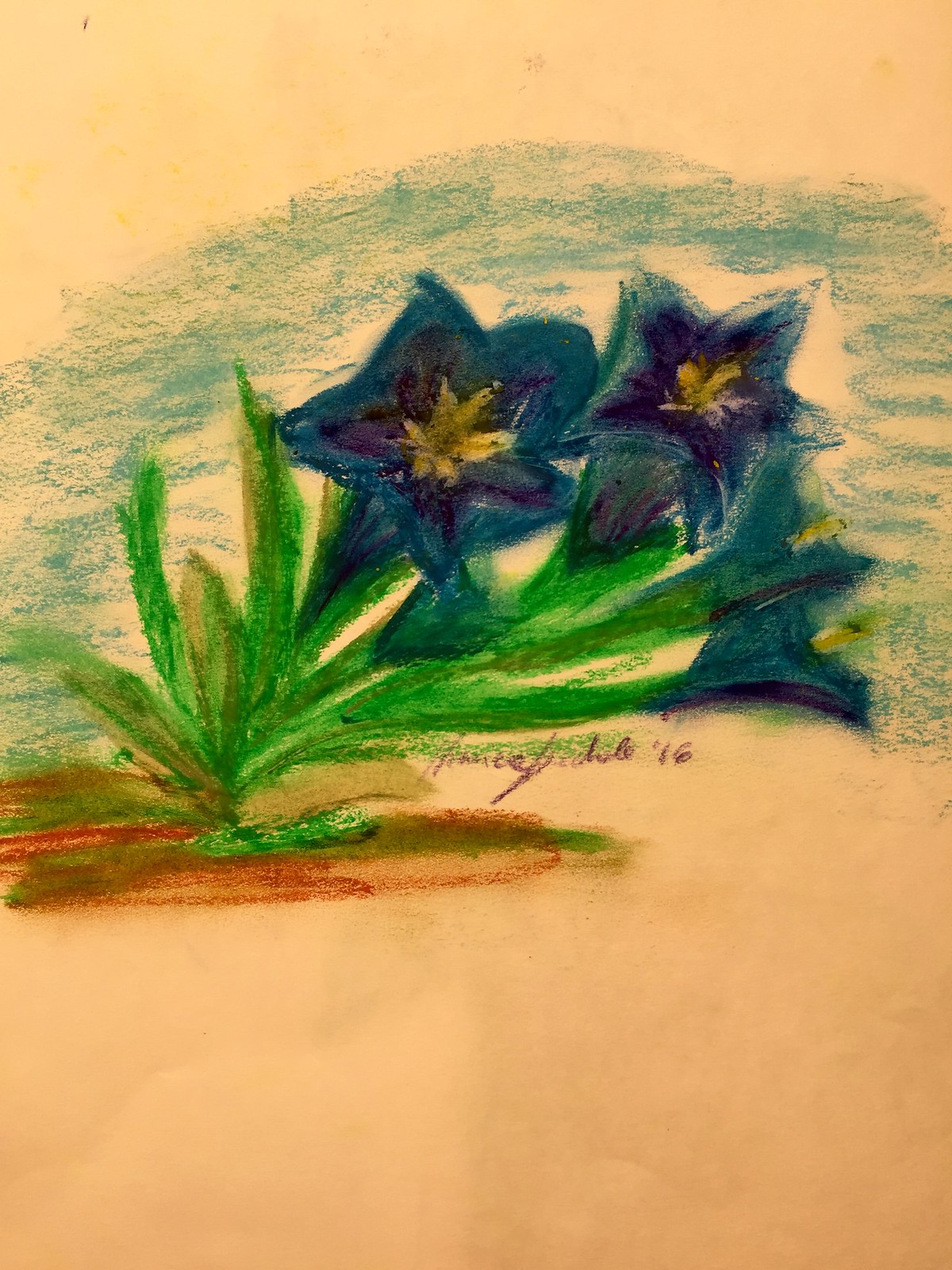This detailed drawing, likely crafted with crayons or pastels, features three prominent, deep blue star-shaped flowers, each with yellow centers, and includes shades of purple towards the middle. The flowers, which are somewhat unique in their coloration, have extra points extending from their petals and appear to be sweeping off to the right of the image. The plant's long, thin green leaves occasionally curve horizontally, creating a dynamic composition. 

The background is a mix of light orange-peach and scattered blue areas, which may represent the sky or a body of water. The base of the plant features brown and reddish tones, indicative of dirt, with some shadowing beneath the flowers adding depth to the image. The paper appears tan or brown with an overall dirty or intentionally shaded texture, and is slightly crinkly.

A signature, although difficult to read, is positioned towards the bottom of the image in purple, likely dating the artwork to 2016, marked with '16. Overall, the image captures a delicate balance of natural elements and artistic flair with its vibrant hues and textured background.